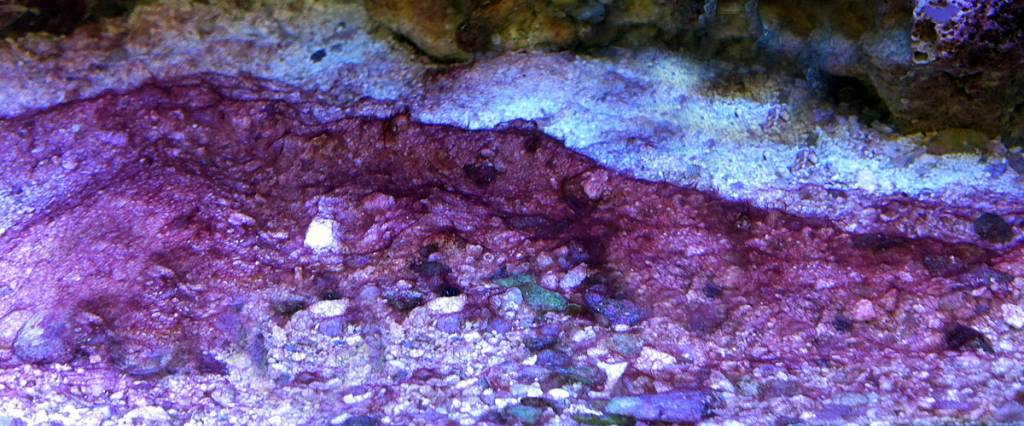The image is an up-close view of a geode that has been cut open, revealing the intricate crystal formations inside. The outer edge of the geode retains its rough, gray rock exterior, transitioning to a lighter band of white that has hints of bluish hues. Central to the image is a rich, dark purple cluster of amethyst crystals, shimmering under bright light. The bottom half of the photo reveals lighter colors again, with specks of aquamarine, blue, and white intricacies within the formation. The overall scene is accentuated by reflective light that gives the crystals a red hue in certain spots, blending with the natural purple and pink tones. The cavernous rock formation inside the geode displays various shapes and sizes, creating an almost otherworldly landscape with holes and unique textures.